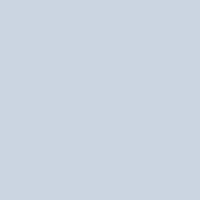The image depicts a light gray, perfectly square box with no additional features such as text, borders, buttons, or icons. The box, rendered in a minimalist style, appears centered within a rectangular frame, which suggests it may be part of a webpage displayed on a mobile device, most likely a smartphone given the vertical orientation. The simplicity and lack of any contextual elements hint at either a design element or a placeholder in a digital interface.